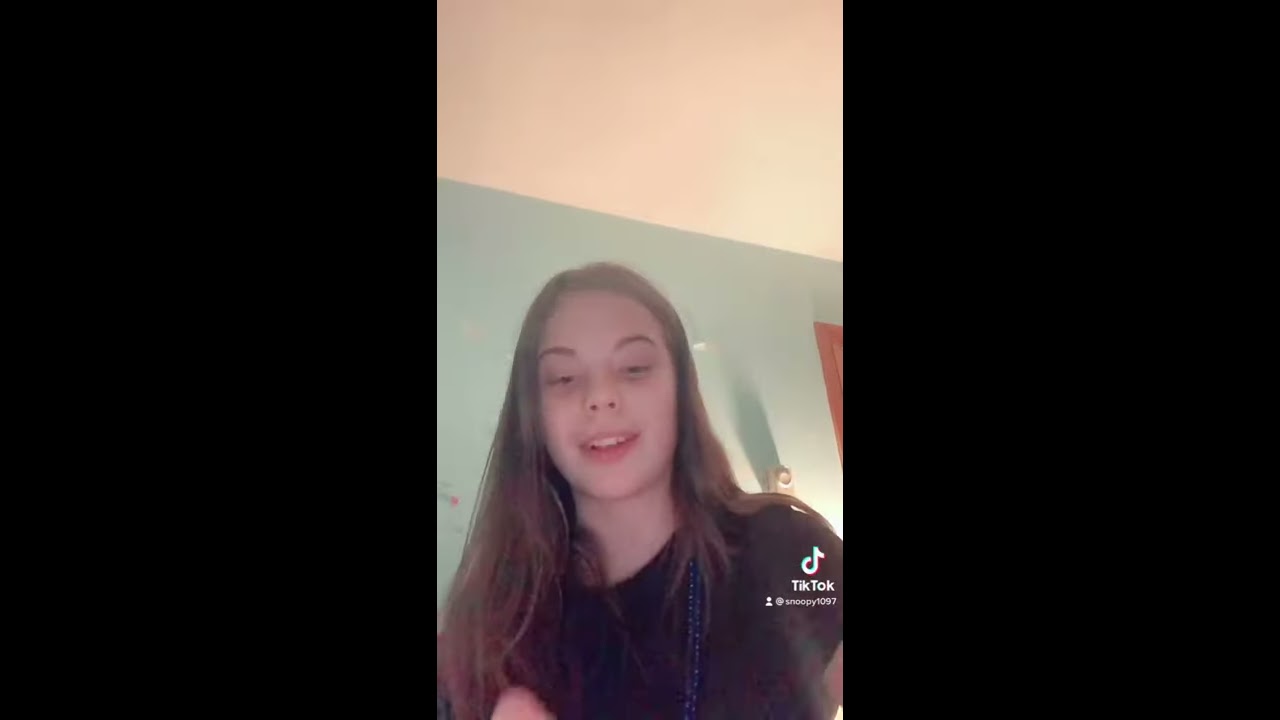This vertical still frame from a TikTok video features a young girl, likely a teenager, with long black hair, wearing a black t-shirt and a blue lanyard around her neck. She is centered in the frame, facing the camera but looking down and smiling, possibly speaking. The TikTok logo and her username, Snoopy1097, are prominently displayed at the bottom right of the image. The background reveals a white ceiling and a light green wall, with the hint of a brown door to the right and a possible thermostat or light dial behind her left shoulder. The setting appears to be an indoor room.